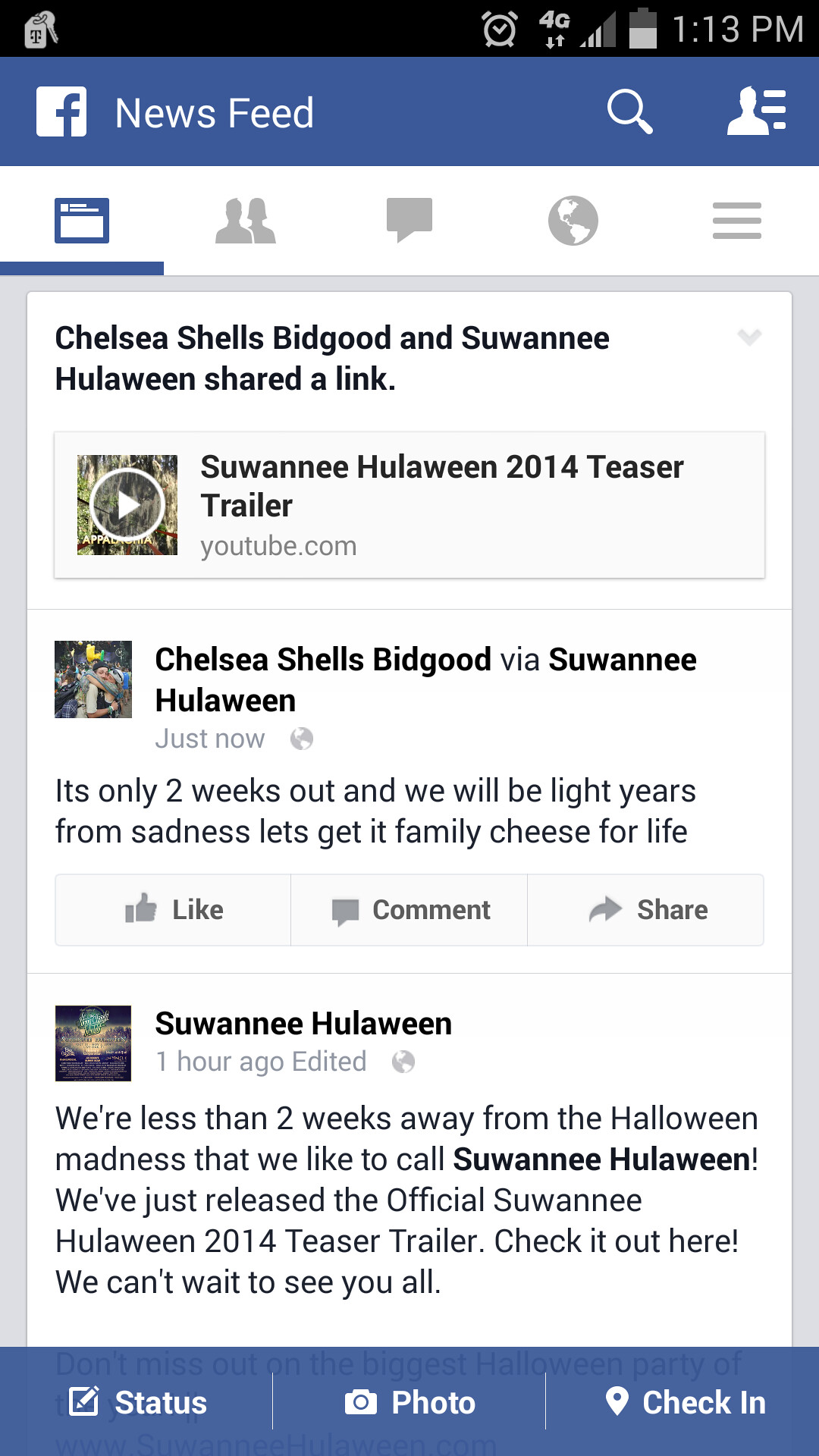The image is a detailed screenshot of a Facebook feed taken from a cell phone, likely an Android device, while the user was browsing the Facebook app. At the very top, the black bar shows various icons in white, including the time of 1:13 p.m., indicators for an alarm clock, 4G connectivity with arrows, cellular bars, battery level, and a key on a keyring. Below that, a blue bar with white text displays the Facebook logo on the top left, the words "News Feed," a magnifying glass, a silhouette of a person, and three lines indicating a menu.

In the main feed, you see posts with typical Facebook interaction options like "like," "comment," and "share." Prominently displayed is a post about Suwannee Huluween, mentioning that it is only two weeks away and promising to transport attendees "light years from sadness." The post also includes a call to action with "Let's get it family, cheese for life." Another part of the post states that the official Suwannee Huluween 2014 teaser trailer has been released, inviting users to check it out with an enthusiastic "We can't wait to see you all."

The image features a color scheme dominated by blue, white, black, green, and gray, and the layout takes up the entire screenshot, clearly indicating it was taken while the user engaged with their Facebook app. The bottom of the screen displays options for status updates, photo uploads, and check-ins, completing the snapshot of the user’s mobile experience.